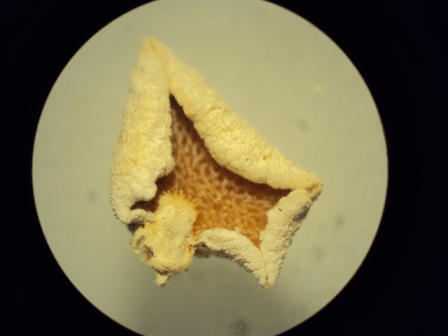This photograph features a semi-close-up image with a dark, black background, highlighting a central circular object that resembles the moon, creating an overall stark contrast. The central circle is a light gray or white, adorned with subtle gray dots scattered across its surface. The subject within this circle evokes images of complex organic material. Its form is intricate and somewhat ambiguous, variously described as resembling a brain, coral, or even tissue seen through a microscope. The structure has a mix of cream, brown, and yellowish hues, giving it a veiny, textured appearance. The outer regions of this unknown entity are cream and white, transitioning to a more yellowish tone towards the center, which bears a web-like or membrane network in shades of light orange and reddish-orange. The photograph has no text or people, and the corners of the image appear folded or curled inward, making the overall form somewhat contained within the rectangular frame of the photograph.